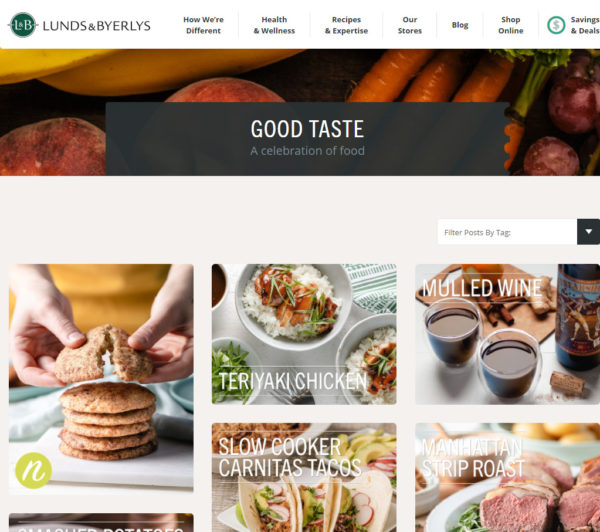A detailed caption for the given image could be as follows:

"A promotional advertisement for Lunds & Byerlys, featuring their signature green circle logo with 'L&B' at the top, surrounded by a white border. The text 'Lunds & Byerlys' and the motto 'How We're Different' are displayed prominently below. Despite being blurry and a bit small, the message 'Health and Wellness' is discernible. Further sections include links like 'Recipes and Expertise,' 'Our Stores,' and 'Shop Online.' The visual display includes fresh produce such as potatoes, carrots, onions, and bananas. A gray box with the tagline 'Good Taste, A Celebration of Food' precedes a series of food images. On the left, there's a close-up of a stack of cookies with someone breaking one in half. To the right, a delicious bowl of teriyaki chicken includes rice and vegetables. Below that, the text 'Slow Cooker Carnitas Tacos' is displayed next to an image of the dish. Adjacent to the carnitas tacos, there's a mention of 'Mulled Wine,' followed by the title 'Marinated Strip Roast' at the very bottom."